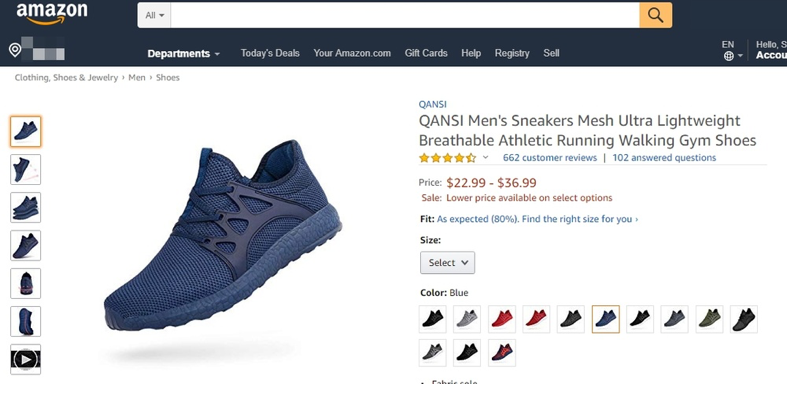This is a detailed caption for the described image:

"A screenshot of the Amazon website showcasing a product listing. At the very top, there is a black header with the Amazon logo on the upper left. The logo is in white, accompanied by a distinctive yellow smile with an arrow beneath it. In the center of the header, there is a search bar labeled 'All' with a magnifying glass icon on its right side. Below the search bar, several navigation sections are visible, including Departments, Today's Deals, Your Amazon.com, Gift Cards, Help, Registry, and Sell.

In the main white area of the webpage, a black sneaker is prominently displayed. To the left of the sneaker, there are thumbnail images offering various views of the shoe, with the top thumbnail highlighted in yellow. The sneaker is positioned with its toe pointing downward and heel upward.

To the right of the main shoe image, product details are provided under the title 'Kwanzee.' The full description reads 'Kwanzee Men's Sneakers, Mesh, Ultra Lightweight, Breathable, Athletic Running, Walking Gym Shoes.' The product has received a rating of four and a half stars from 662 customer reviews, and there are 102 answered questions. The price range is listed as $22.99 to $36.99, with a note that a lower price is available on select options. An '80% Fit As Expected' metric is indicated, along with a prompt to 'Find the right size for you.' There is a size selection dropdown menu visible. The mouse cursor is highlighting the black shoe option, suggesting the user is in the process of making a selection."